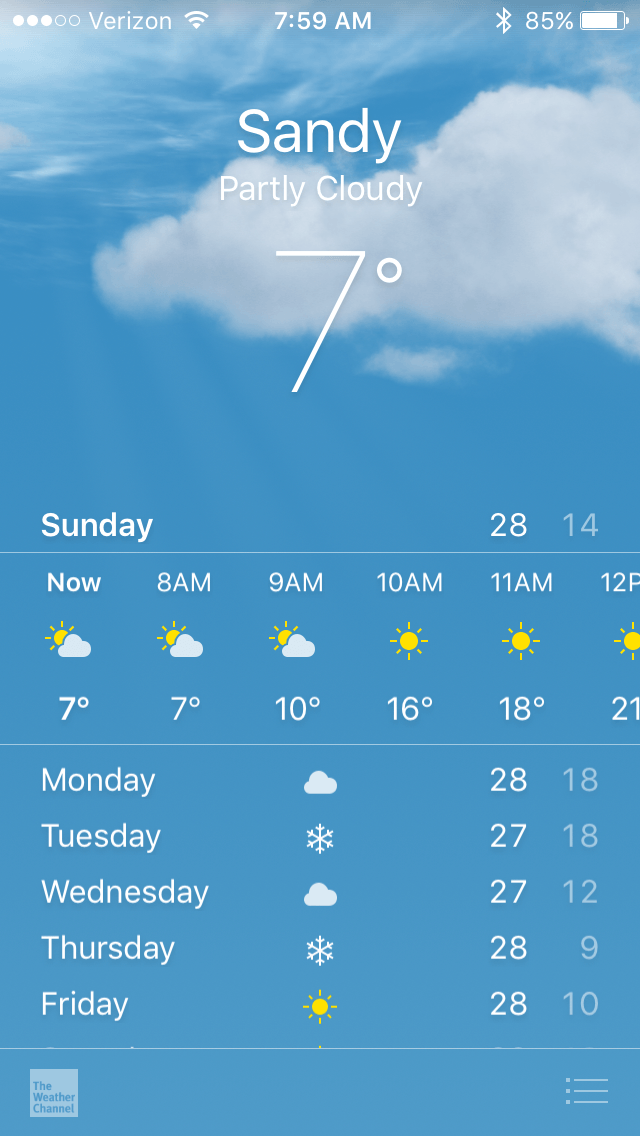This image is a screenshot captured from a smartphone, displaying a detailed weather forecast and other interface elements. The top of the screen shows the status bar with the carrier name "Verizon", the current time "7:59 AM", an active Bluetooth indicator, and a battery life of 85%. The background is a gradient of sky blue with white, fluffy clouds. Across this background, white text provides the current weather conditions: "Sandy, partly cloudy, 7 degrees".

Below, the day "Sunday" is prominently displayed along with the high and low temperatures "28" and "14" respectively. This is followed by a detailed hourly forecast:
- "Now: partly cloudy, 7 degrees"
- "8 AM: partly cloudy, 7 degrees"
- "9 AM: partly cloudy, 10 degrees"
- "10 AM: sunny, 16 degrees"
- "11 AM: sunny, 18 degrees"
- "12 PM: sunny, 21 degrees"

A white line separates the hourly details from the weekly forecast, where each day's condition and temperature range are listed:
- "Monday: cloudy, high of 28, low of 14"
- "Tuesday: snowy, high of 27, low of 18"
- "Wednesday: cloudy, high of 27, low of 12"
- "Thursday: snowy, high of 28, low of 9"
- "Friday: sunny, high of 28, low of 10"

Another white line marks the end of this section. In the bottom corners of the screen, the emblem of The Weather Channel appears on the left, while three horizontal lines for more information are located on the right.